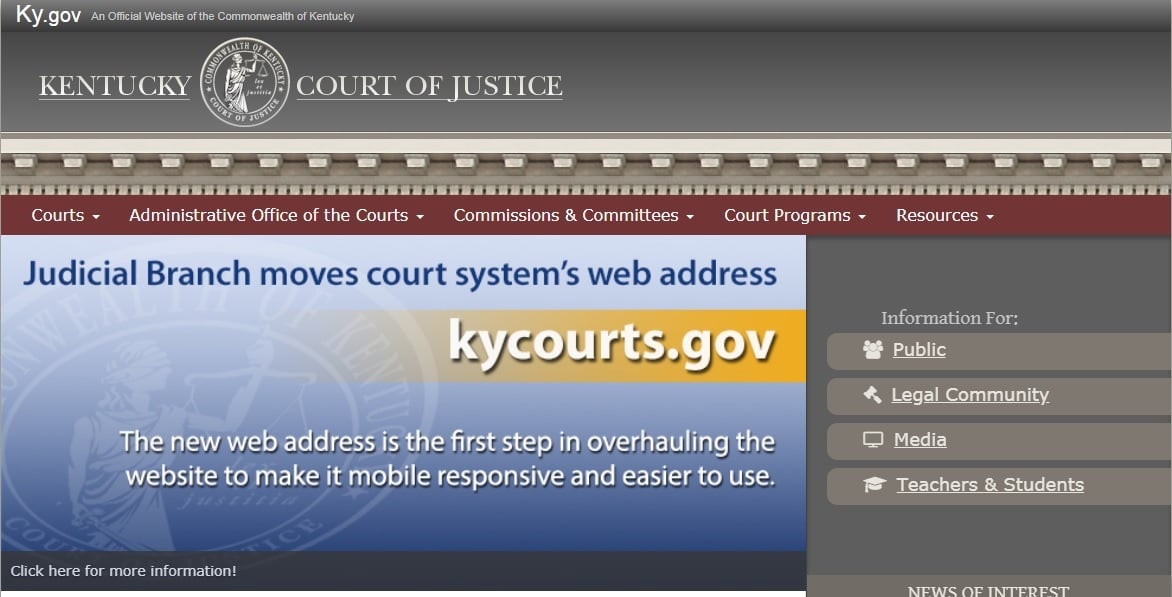The image is a detailed partial screenshot of the official website of the Commonwealth of Kentucky, ky.gov. At the top, the page features the seal of the Kentucky Court of Justice prominently. The header is followed by a set of burgundy navigation tabs with drop-down arrows for various sections: "Courts," "Administrative Office of the Courts," "Commissions and Committees," "Court Programs," and "Resources."

The main body showcases an article announcing the judicial branch's decision to update the court system's web address to kycourts.gov. The article notes that this change is part of a broader effort to make the website more mobile-responsive and user-friendly.

To the right of the main content is a gray sidebar featuring a list titled "Information for," which serves as a guide for different groups: the public, the legal community, the media, teachers, and students. Below this section, there is a "News of Interest" area with a CTA (call-to-action) prompting users to "click here for more information."